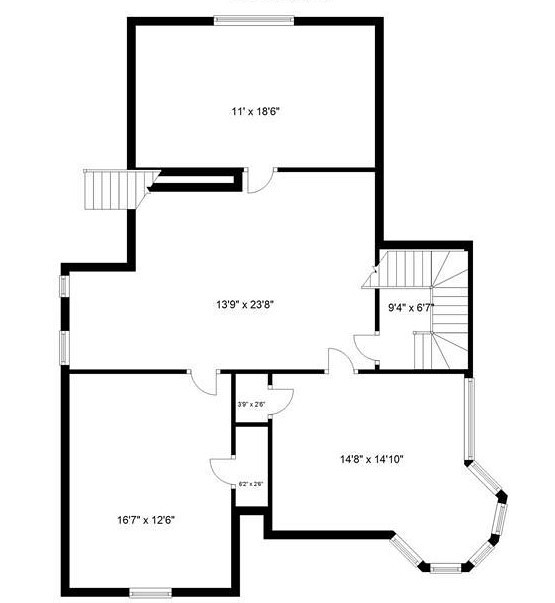This blueprint depicts the upstairs layout of a house, featuring a central common room surrounded by three bedrooms. The common room, measuring 13 feet 9 inches by 23 feet 8 inches, is centrally located with two sets of stairs leading downward situated on either side. 

Flanking the bottom of the common room are two bedrooms: the left bedroom measures 16 feet by 12 feet, and the right bedroom is 14 feet by 14 feet, each equipped with its own closet. Positioned above the common room is the third bedroom, which measures 11 feet by 18 feet. 

Additionally, the lower right-hand bedroom includes a distinctive architectural element—a cupola. The blueprint is rendered in black ink on a white background, providing a clear and detailed plan of the upper floor.